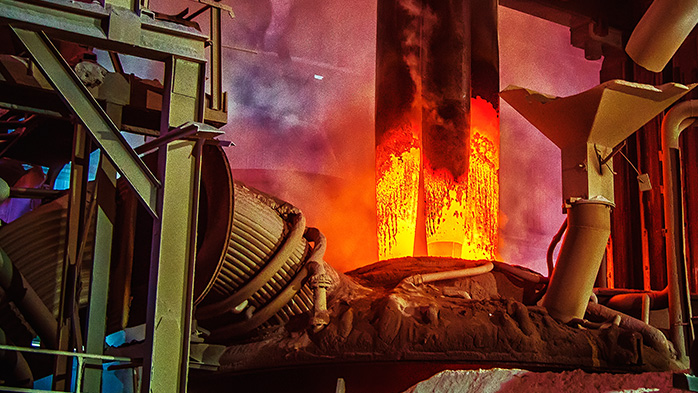The image captures an intense scene within an industrial setting, reminiscent of a frame from a movie but grounded in reality. Central to the composition, a massive mound anchors the scene, from which multiple tubes and chutes emerge. These tubes appear to be spewing vibrant, fiery substances like molten metal or lava, in shades of yellow, orange, and red, with dense plumes of smoke and steam billowing above. On the left side, the structure is framed by large metal scaffolding, painted gray or green, complete with railings and surrounded by a network of pipes. Among these pipes is a prominent ridged tube that extends off-screen, encircled by various round rings. This industrial tableau, with its combination of molten materials and complex machinery, teems with raw energy and the harsh beauty of industrial processes.